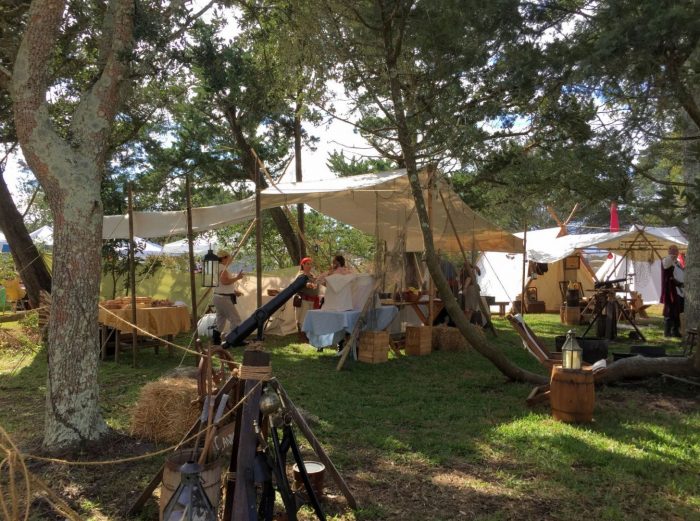This bustling color photograph captures a lively campground nestled within the woods, suggestive of a role-playing event or historical reenactment. In the foreground, a tall tree trunk stands on the left, accompanied by a bale of hay. Nearby, a wooden tripod, possibly for a campfire, and some dark-colored lanterns atop wooden barrels draw your attention. The grassy area is dotted with various camping gear and a few people. Under a central canvas canopy, two or three individuals, dressed in light-colored clothes with handkerchiefs tied around their heads, are seen milling about tables.

Beyond this main canopy, which stands about 8 to 10 feet off the ground and has no sides, there's another similar structure off to the right. Scattered around this camp, you'll find wooden crates, additional hay bales, and more lanterns. The green grass, showing hints of yellowing, lies mostly in shadow due to the elongated trees casting their late-day shade.

The background is a dense forest of green-leafed trees with brown trunks and some sporadic white and green hues on their bark. The sky peeking through the treetops is a light blue interspersed with white, further indicating the onset of evening. People in tan outfits, some with hats, are visible under the canopies, standing or sitting on brown chairs. A white cloth-covered table holds a prominent spot nearby, with two wooden boxes in front and a metal object with tan ropes and nearby hay completing the rustic scene.